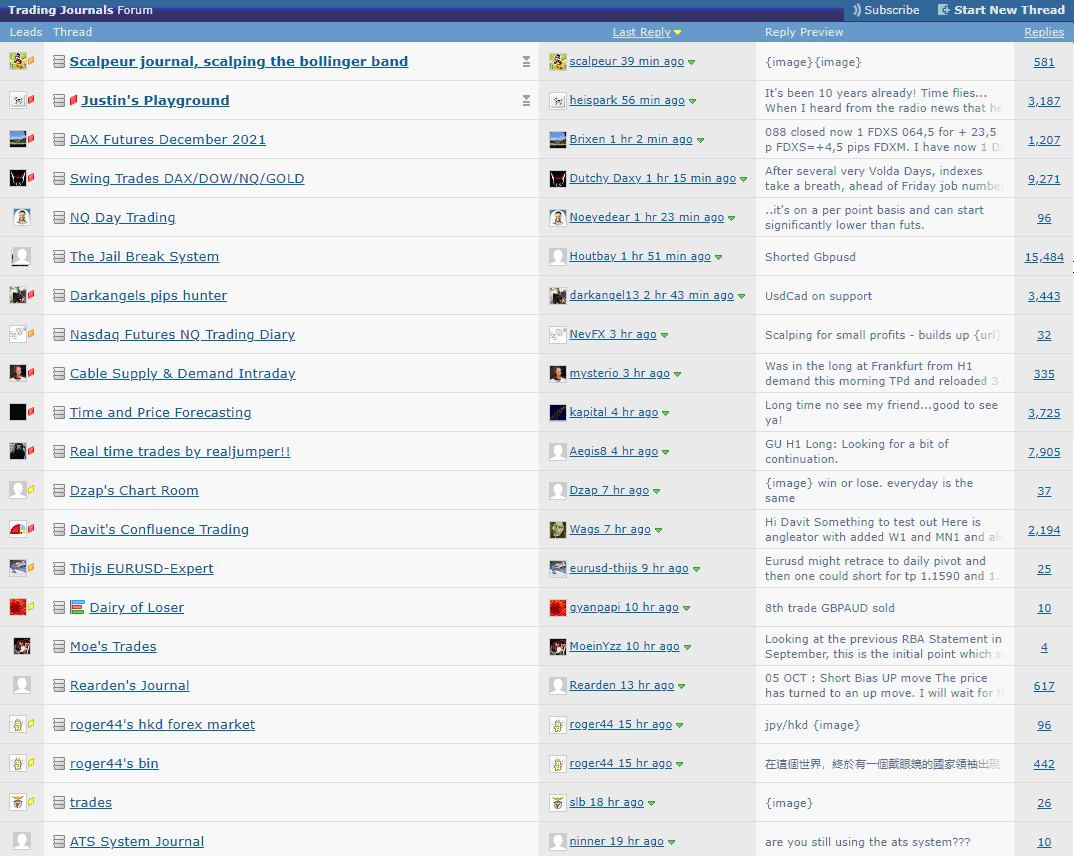The image captures the interface of a Trading Journals Forum. In the top left corner, the forum's title is displayed in blue: "Trading Journals Forum." On the top right, two buttons are visible: "Subscribe" and "Start New Thread." 

Below this header section, the forum's content is organized into three columns. The first row features a thread titled "A Scalper's Journal: Scalping the Bollinger Band," written in darker blue text. Each column is titled as follows: "Leads" (which likely displays an image of the user who started the thread), "Thread," "Last Reply," "Reply Preview," and "Replies." 

Several threads are listed underneath, each initiated and updated by various users. Notable thread titles include:

- Justin's Playground
- DAX Futures, December 2021
- Swing Trades: DAX/DOW/NQ/Gold
- NQ Day Trading
- The Jailbreak System
- Dark Angel's Pips Hunter
- Nasdaq Futures Note: NQ Trading Diary

Each thread’s listing provides details such as the name of the last person who replied, the time elapsed since that reply, a snippet of the latest message in the Reply Preview section, and the total number of replies. This detailed layout allows users to navigate through active discussions, follow updates closely, and participate in trading-related conversations efficiently.